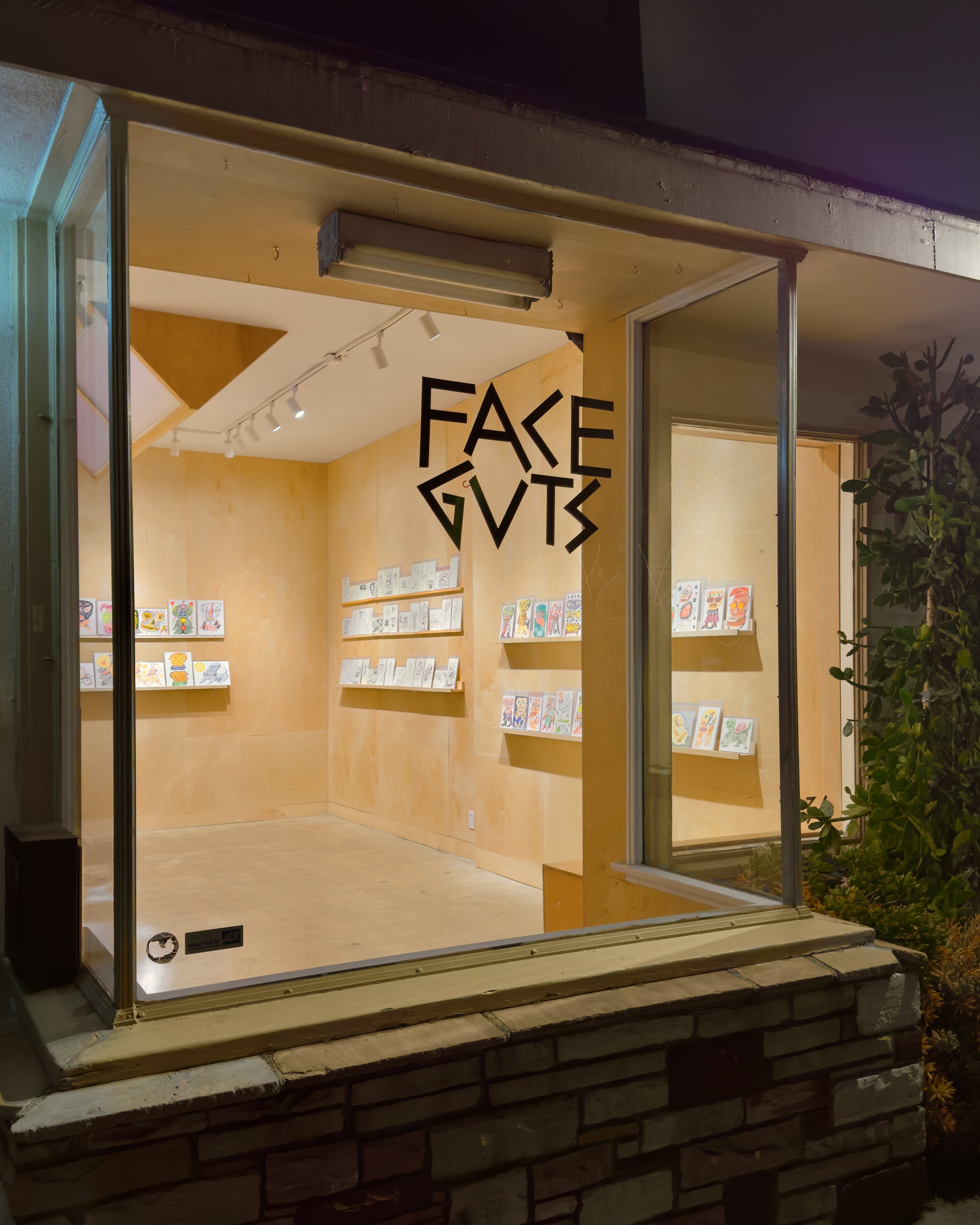In this image, we see the exterior of a storefront, potentially an art gallery, with a large, square window framed by multicolored bricks at the bottom. The window is illuminated despite the nighttime setting, showcasing black, stylized, edgy text that reads "Face Guts." Inside, the walls and floor are light brown, giving the interior a warm, inviting feel, while the ceiling is white with overhanging lights directed toward the walls, highlighting the displays. The walls feature floating shelves adorned with various 8x10 edgy illustrations. To the right of the storefront, a green plant with a few bushes enhances the exterior's natural feel.